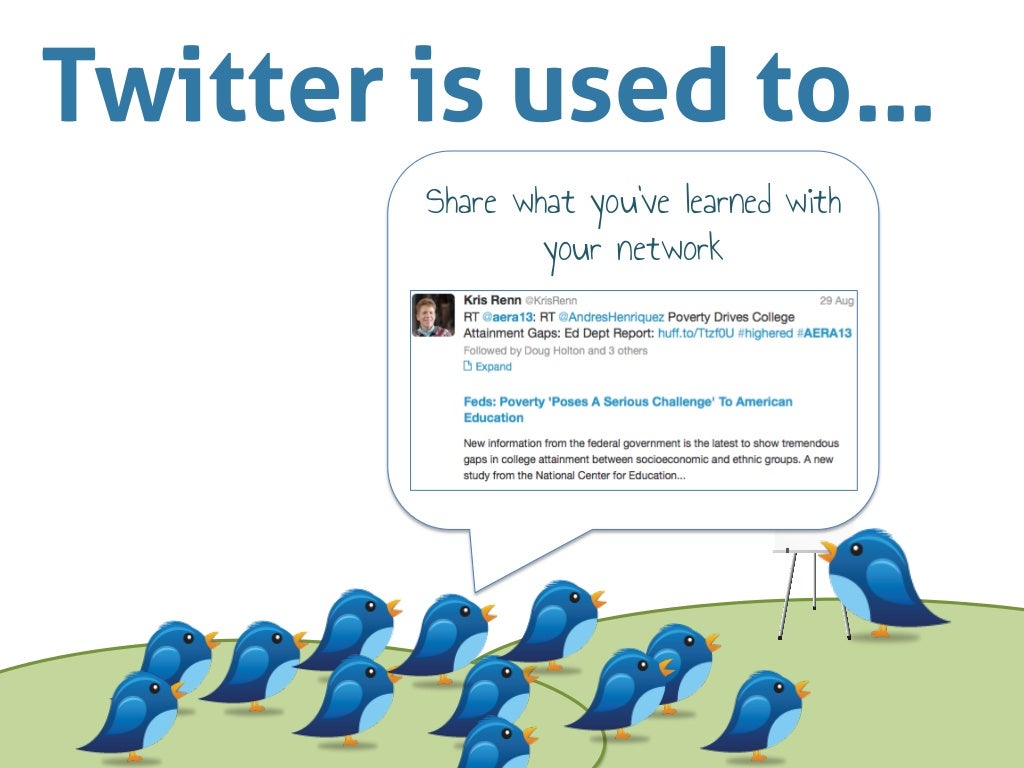The image showcases a cartoon-style artwork set against a white background. Bold blue text at the top reads, "Twitter is used to...". The scene depicts a green grassy landscape with a blue bird facing left standing beside a whiteboard-like podium. The bird appears to be presenting information to an audience of smaller blue birds, all facing the right-hand side of the image. A thought bubble above the presenting bird contains the text: 

"Share what you've learned with your network. Chris Ren RT @AERA13 RT @AndreasHenriquez Poverty drives college attainment gaps EV Department reports Huff.to. Fed: Poverty poses a serious challenge to America's education. New information from the federal government is the latest to show tremendous gaps in college attainment between socioeconomic and ethnic groups. A new study from the National Center of Education."

This detailed scene effectively conveys the educational message about the impact of poverty on college attainment through an engaging and visual format.